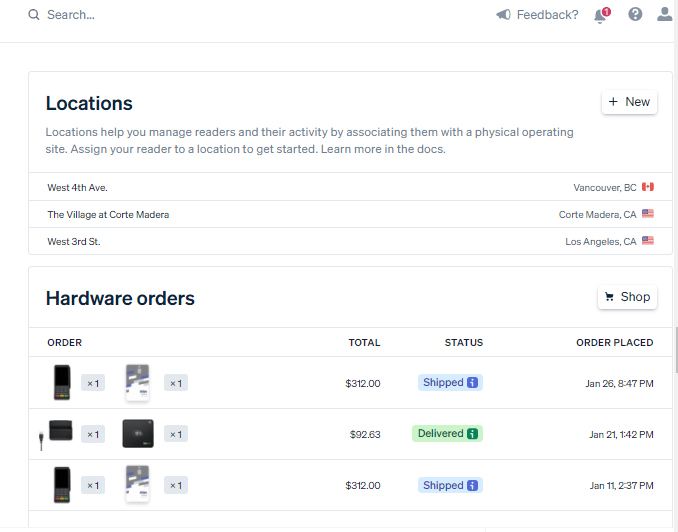The user interface displays several key elements, including a search bar, feedback option, a notification icon with a red circle indicating one new notification, a gray circle featuring a question mark for help, and a profile icon. The section on "Locations" helps users manage readers and their activities by associating them with physical operating sites. Assigning a reader to a location is the first step, with additional details available in the documentation.

A prominent "New" button in black lies within a rectangle, providing options to create new entries. Below, specific locations are listed:

1. **West 4th Ave, Vancouver, B.C., Canada:** Identified with the Canadian flag.
2. **The Village, Corte Madera, C.A., USA:** Identified with the U.S. flag.
3. **West 3rd Street, Los Angeles, C.A., USA:** Also marked with the U.S. flag.

The "Hardware Orders" section displays a shop icon resembling a buggy. The order details include the total number of items, their status, and the date and time the order was placed:

1. **First Order:**
   - 1 item described as "phone"
   - A pictogram of a car
   - Order number: 312
   - Status: "Shipped" in blue
   - Order placed: January 26th, at 8:47 PM

2. **Second Order:**
   - 1 item described as "charger"
   - No additional details provided

This detailed interface allows efficient navigation and management of various aspects related to locations and hardware orders.